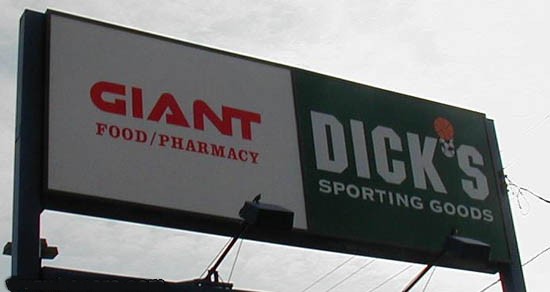This image captures a large billboard framed and supported by sturdy green metal posts. The sign itself is divided into two distinct sections. The left portion features a white background with bold red text that reads "GIANT FOOD PHARMACY." The right section has a green background with "DICK'S SPORTING GOODS" prominently displayed in large white letters. Notably, the apostrophe in "Dick's" is creatively designed using an orange basketball and a black and white soccer ball. Supporting poles are visible behind the sign, adding stability, and several power lines can be seen in the background. The sky overhead is a uniform light gray, devoid of any other colors or patterns.